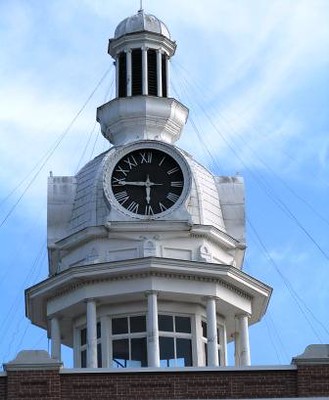This photograph captures a striking clock tower perched atop a red brick building. The base of the tower is a brown brick octagon with elegant white pillars at each corner. Above this, a dome structure supports a large black clock face, which features prominent white Roman numerals and hands, displaying the time as quarter to six. The section with the clock is crafted from white wood. This clock face encompasses the entire upper part of the tower and is framed by a white ledge that further elevates the structure. At the top of the clock portion, there's another smaller, white domed segment on top of the ledge, adding an intricate finishing touch with black in the middle and more white pillars. The entire tower stands tall against a backdrop of a bright blue sky adorned with soft white clouds. The photograph emphasizes the clock tower's architectural details, highlighting its towering presence and the contrasting colors that make it an eye-catching edifice.